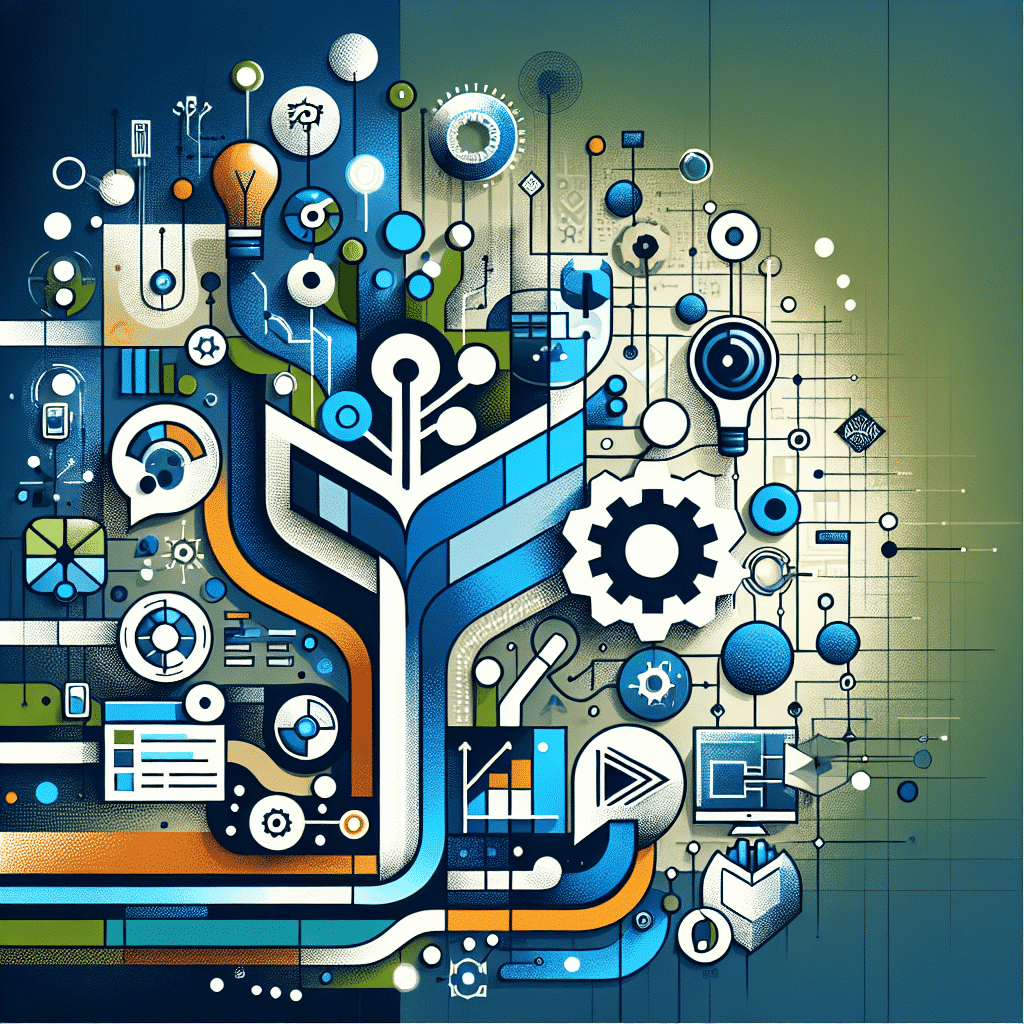This image is a vibrant and intricate piece of digital artwork characterized by its abstract, geometric style. Predominantly colored in shades of blue and green, with accents of orange, white, and black, the scene is busy and densely packed with various interconnected elements. It features an array of semi-familiar icons such as modern light bulbs, gear signs reminiscent of computer settings, graphs, pie charts, and play button symbols, all rendered in a cartoony, stylized manner. The artwork is dominated by round shapes and thin rectangular lines that link the different components together, creating an impression of interconnectedness, perhaps suggesting the flow and generation of energy. The absence of text invites viewers to interpret the complex interplay of mechanisms and symbols, allowing for personal perception and imagination. Overall, the piece blends a technical, contemporary aesthetic with bright, engaging colors and dynamic composition.